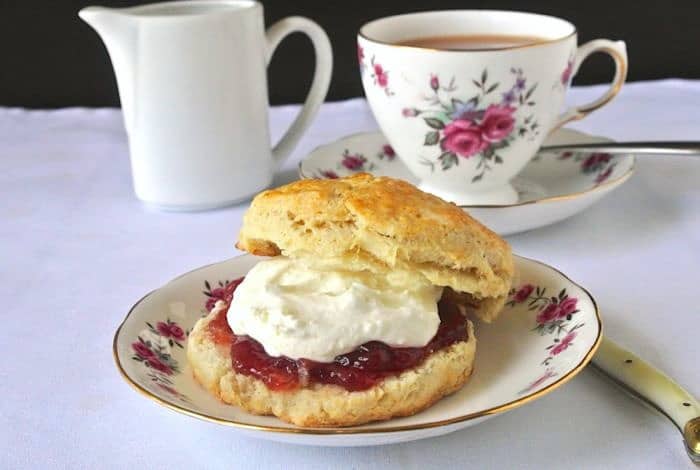In the image, an elegantly set table showcases a delightful breakfast arrangement. Central to the scene is a split biscuit filled with a layer of jam and a dollop of cream or whipped butter, meticulously placed on a fancy plate adorned with pink and purple flowers and intricate gold detailing around the edge. Accompanying the biscuit is a matching teacup filled with coffee or tea, perched on a similarly decorated saucer. A small silver spoon leans against the saucer, while a plain white creamer sits nearby, ready for use. All of this is set against a backdrop of a pristine white tablecloth, with a stark contrast provided by a dark, possibly black, background, making the vibrant details and colors of the dishware and food pop out from the image.